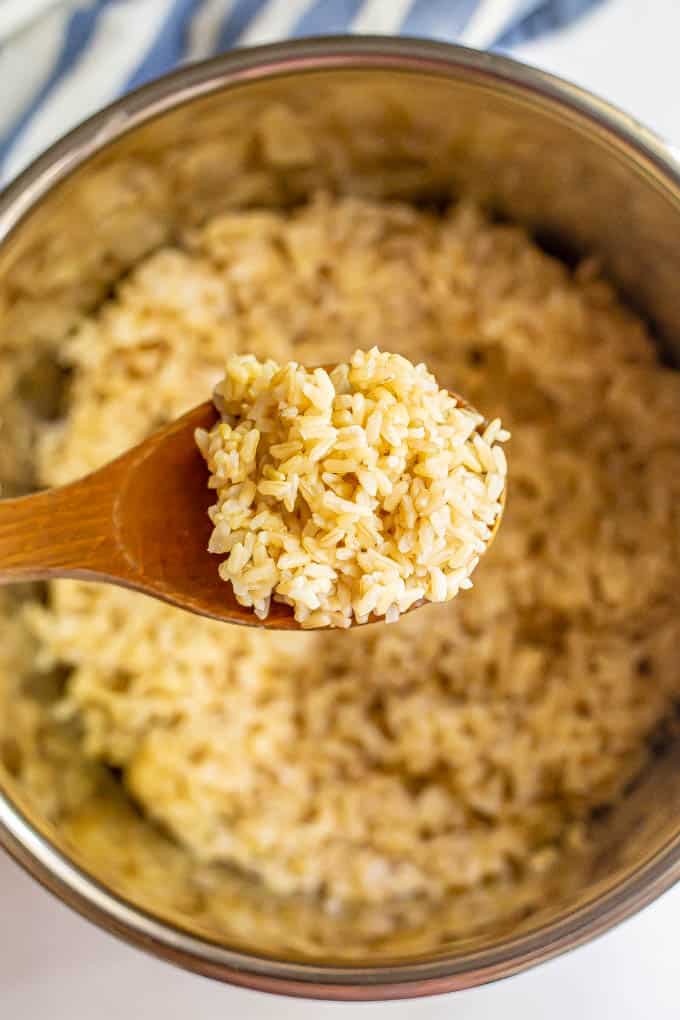The photograph features a close-up of a wooden spoon filled with cooked brown rice, highlighted in clear daylight. The rice, with its thicker, chewier texture and light beige color, is densely packed on the spoon. Below the spoon, a reflective, metallic bowl about halfway full of brown rice serves as the backdrop. The bowl's surface shows the clustering of the rice grains, enhancing the depiction of the cooked rice's texture. The spoon appears to be held from a left-hand perspective, adding a natural, human element to the composition.